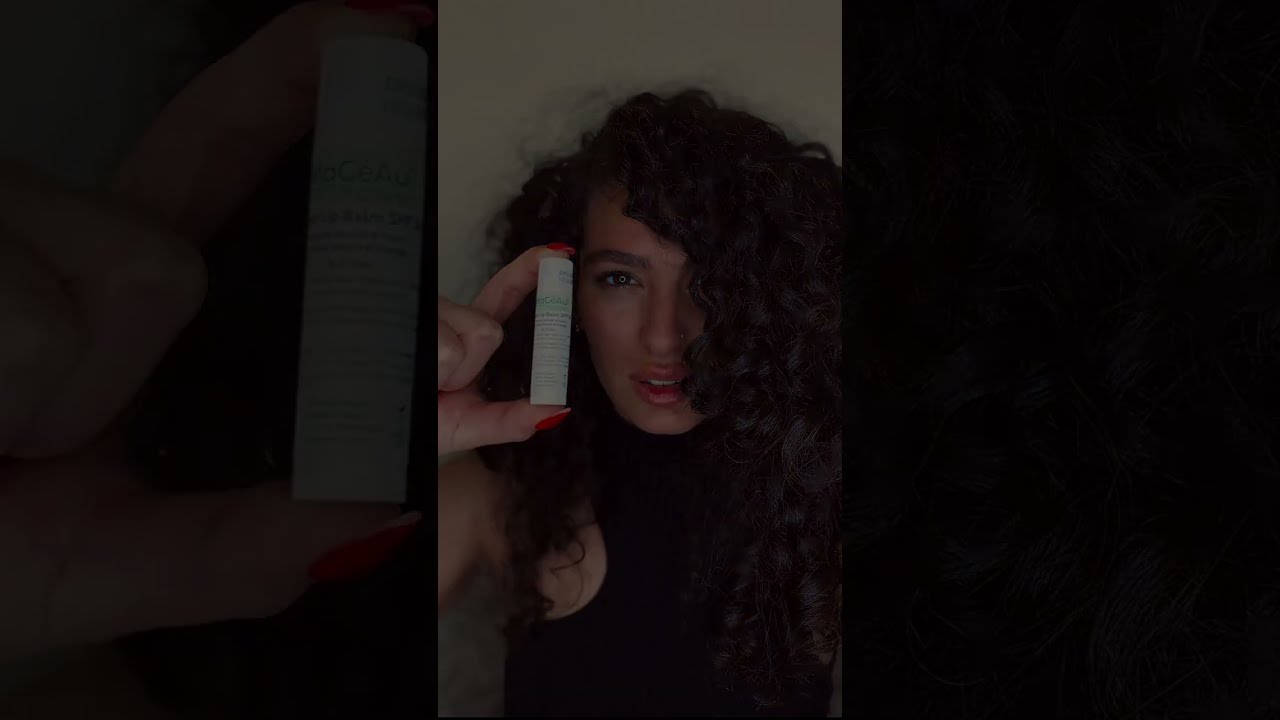In this detailed close-up image, a woman is centered against a white wall, holding a small, light gray tube with extensive writing on it between her thumb and index finger. Though the writing is not legible, the tube resembles a cosmetic product or personal item. The woman, adorned in noticeable makeup, boasts thick eyebrows and lipstick that accentuates her brown eyes. Her long, flowing, black curly hair cascades down to mid-chest and partially obscures one side of her face. She wears a black, sleeveless shirt. Her fingernails, painted a striking red, contrast sharply with the dark tones of her attire and surroundings. The image is framed by large, black rectangles on either side, and the overall scene is dimly lit, adding a dramatic focus on both her facial features and the tube she presents.